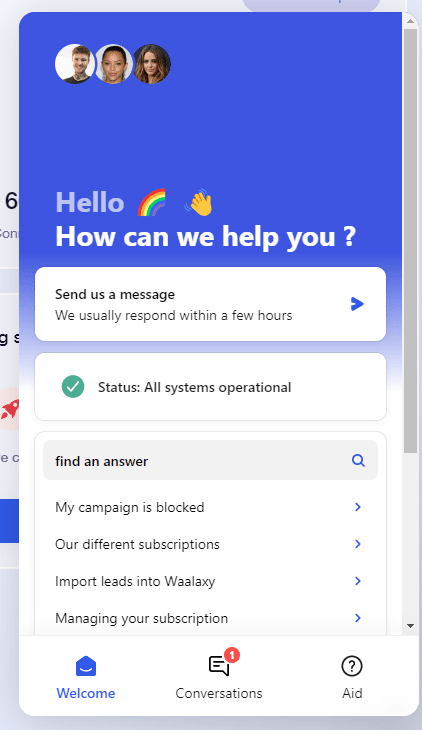In the presented image, the top half of the background is shaded in a vibrant blue. Positioned in the top left corner are three profile icons, arranged horizontally: one male profile icon flanked by two female profile icons. Below these icons, the text "Hello," is prominently displayed in white, accompanied by a colorful rainbow image and a cheerful yellow waving hand emoji. The text continues, saying, "Hello, how can we help you?"

Below the blue section, there is a transition to a black background where the white text reads: "Send us a message, we usually respond within a few hours." To the right side of this message, there is a blue button intended for sending messages.

Further down, the background of the interface turns white, forming the search engine area. Here, a status update is shown with the text: "Status: All systems operational." Accompanying this status is a green circle with a tick mark inside, signifying that everything is functioning smoothly.

Underneath this status section, the text "Find an answer" is presented with an adjacent search box. Several suggested inquiries are listed, including "1. My campaign is blocked," and other links such as "Different subscriptions," and "Important link to Wallaxy," with "Manage your subscription" following these suggestions.

At the very bottom of the interface, there are three buttons aligned from left to right. The first button on the left, labeled "Welcome," is highlighted in blue, indicating it's the current selection. The middle button is labeled "Conversation," and it features a red circle with the number one inside, signifying an unread conversation. Lastly, the button on the bottom right displays the number eight and a question mark icon in the center, both of which are black, unlike the "Welcome" button which is blue.